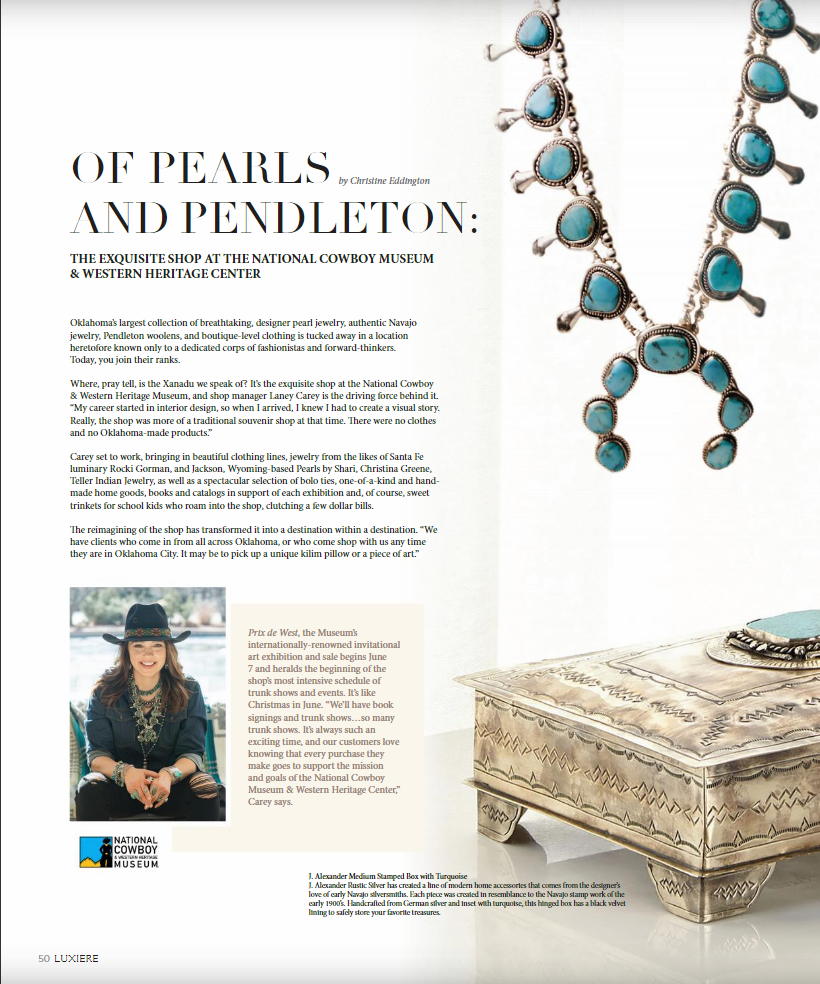The image appears to be an advertisement or article titled "Of Pearls and Pendleton," featuring detailed content about a jewelry collection available at the National Cowboy Museum and Western Heritage Center. The layout is predominantly in white or off-white hues. On the left side of the image, there is a bold headline at the top, "Of Pearls and Pendleton," authored by Christine Eddington. Beneath the headline, an article describes "The Exquisite Shop at the National Cowboy Museum and Western Heritage Center," followed by several paragraphs of text.

An image of the author, Christine Eddington, is positioned below the text. She is seated, adorned in a black cowboy hat and a dark, long-sleeved shirt with the sleeves rolled up to her elbows, paired with dark pants that show fraying at one knee. To her right, a small tan box contains information about the "Prix du West" international art exhibition and sale beginning on June 7th. Below Christine's image, there is a logo featuring a clip art cowboy by a mountain, labeled "National Cowboy Museum."

On the right side of the image, a necklace featuring a blue stone with black specks, held together with metal chains, is prominently displayed. The top half of the necklace is cropped out. Adjacent to the necklace, at the bottom right corner, is a metallic jewelry box with intricate etchings and a matching blue stone on its lid. The bottom of the page includes small, unreadable notes and the mention of "50 L-U-X-I-E-R-E" in the bottom left corner. The overall color scheme includes teal, silver, off-white, black, white, and tan. The image composition combines both real photography and digitally created elements, suggesting a polished, professional layout aimed at emphasizing the unique jewelry collection.